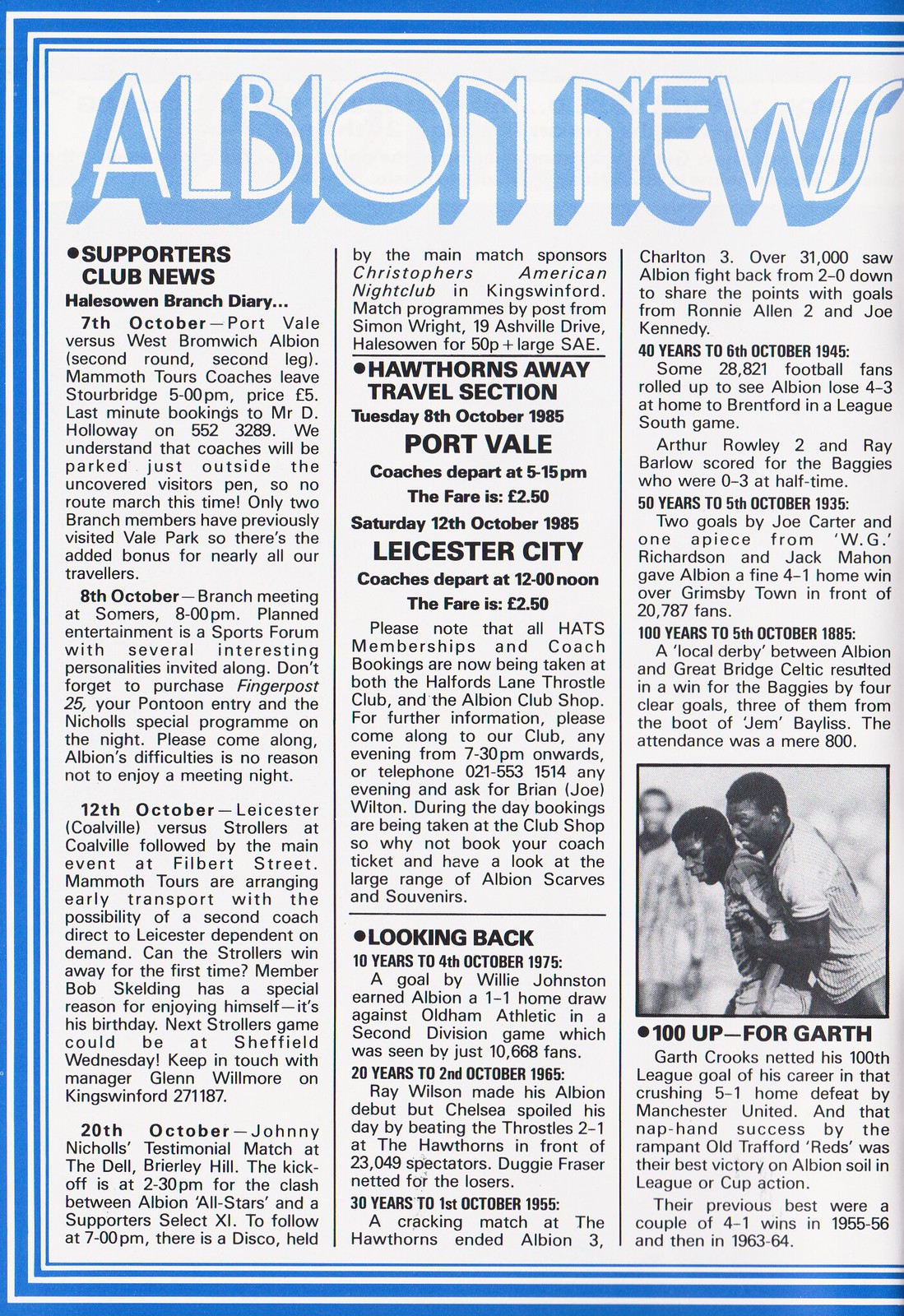The image is a digital scan of an old newspaper page titled "Albion News," characterized by a blue, striped border. Prominently, the page features multiple sections including Supporters Club News, Hill Zone Branch Diary, and Hawthorne's Away Travel Section. The article is centered around several upcoming football events and travel arrangements for supporters.

Key highlights include the announcement for the Port Vale versus West Bromwich Albion match on October 7th, highlighting the second round, second leg. Mammoth Tours will provide coach transport departing from Stourbridge at 5 p.m., with prices set at £5. For last-minute bookings, contact Mr. D. Holloway at 523-289.

Only two Hill Zone branch members have previously visited Vale Park, making this trip a novel experience for most travelers. An additional meeting is scheduled for October 8th at Summers, featuring a sports forum with notable personalities.

Notably, the page mentions Garth Crooks scoring his hundredth career goal during a significant 5-1 home defeat by Manchester United. Additionally, on October 12th, there will be a match involving Leicester City, and transportation for this event departs at noon for a fare of £2.5.

A small black-and-white photograph in the bottom right depicts two football players in a celebratory pose, with another player visible in the background. The travel section also informs that coach bookings and membership inquiries can be made both at the Halsford Lane Throstle Club and the Albion Club Shop, with further contact details provided for convenience. 

In essence, the image captures a vibrant slice of football supporter culture and logistical arrangements from a past era, underscoring the communal spirit and detailed planning involved in following and supporting the beloved sport.